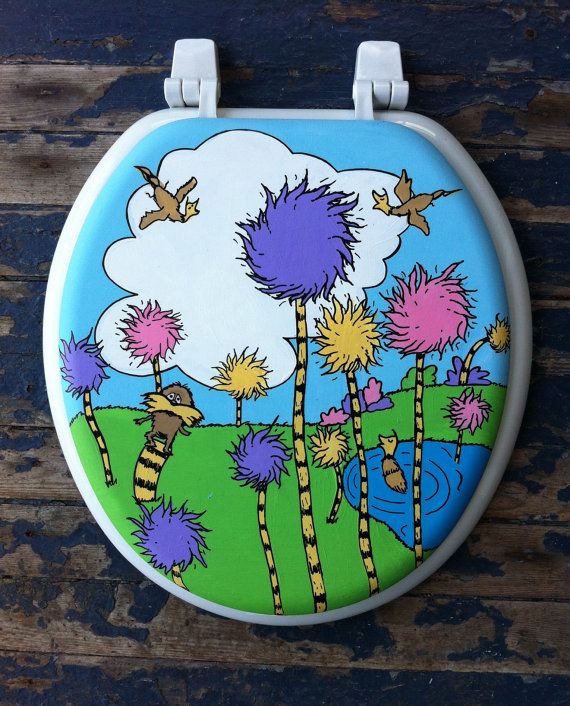This photograph features an unattached toilet seat placed on a rough, worn wooden surface marked with black imperfections, suggesting the paint has eroded over time. The white toilet seat is closed, revealing a vibrant design inspired by a Dr. Seuss scene on the lid. The artwork starts with a bright green grassy field at the bottom, transitioning to a clear blue sky above, punctuated by a single, puffy white cloud outlined in black. Two brown birds with yellow heads soar with their beaks open, pointing skyward, against this backdrop. Emerging from the green are several whimsical trees with yellow and black striped trunks and cotton-like tops in shades of purple, yellow, and pink. A small blue pond appears at the lower right, hosting a two-segmented brown creature with a yellow head, similar to the birds. To the left, atop a tree stump, stands a small brown creature with a prominent yellow mustache and round white eyes with black pupils. This colorful, cartoonish scene brings a playful, storybook quality to an otherwise mundane object.